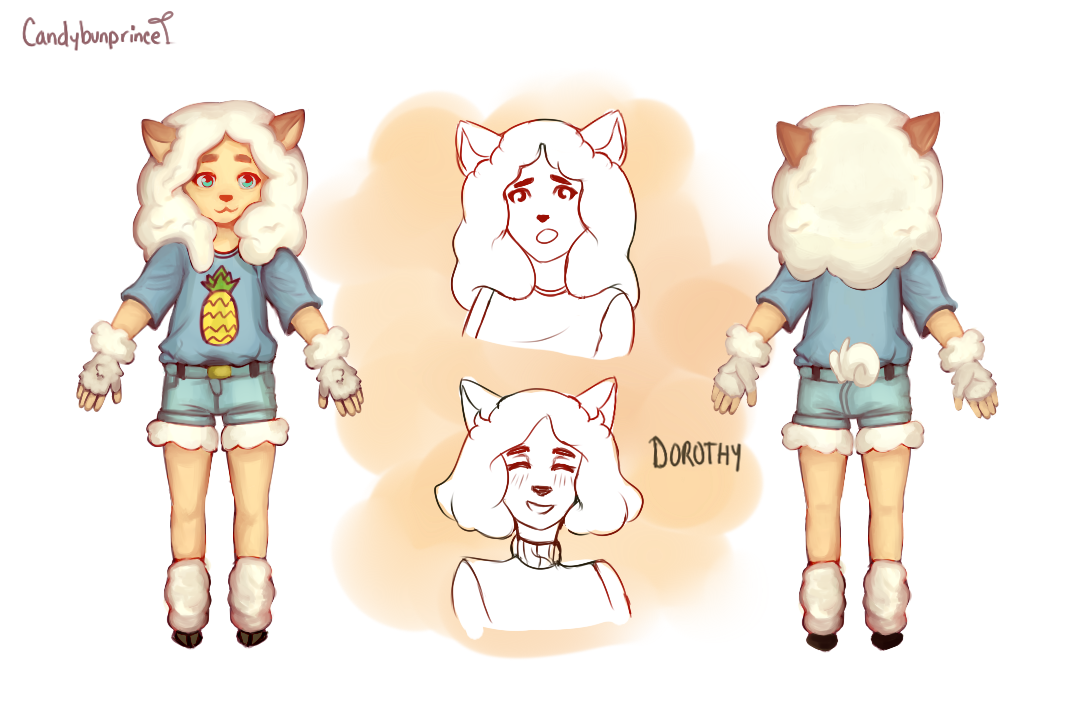The image is a cartoonish drawing, with "Candy Bun Prince" written in the top left corner, decorated with a small leaf design. The central figure is a doll-like character named Dorothy, identified by the pencil text near her on the bottom right. Dorothy has white, fluffy, shoulder-length hair resembling cotton candy, with brown ears protruding from it. Her attire includes a pineapple-printed, mid-length blue t-shirt, and denim shorts with ruffled edges. She is adorned with fingerless gray gloves and pink boots trimmed with white fur. Dorothy's animalistic features include fur around her wrists, ankles, and what appears to be black hooves or cat/lamb-like feet, as well as a fluffy tail visibly protruding from the back view. The image also features two additional smaller drawings of Dorothy in the center, one showing her with a surprised expression and the other with a happy expression. The rear view of Dorothy matches the front, except there is no pineapple decal visible on the shirt.